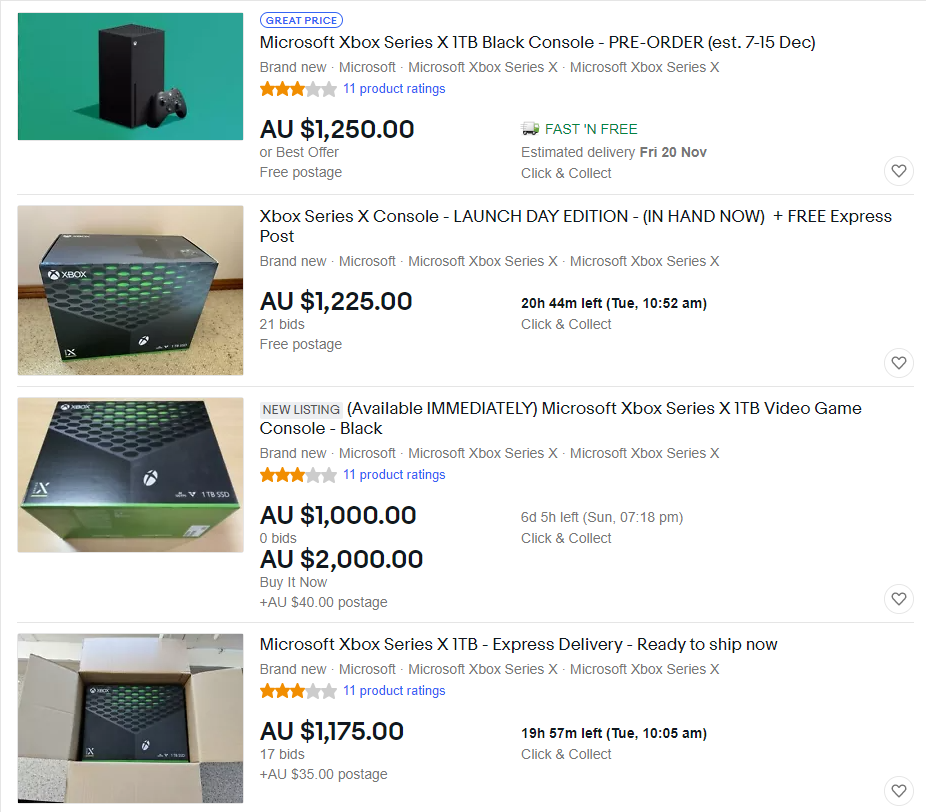In this image, there are listings for four Microsoft Xbox Series X game consoles. The first listing details a Microsoft Xbox Series X, 1TB Black Console priced at $1,250 AUD, with a rating of 3 stars out of 5. The second listing is for an Xbox Series X console, launch day edition, priced at $1,125 AUD, currently receiving 21 bids and with 20 hours and 4 minutes remaining in the auction. The third listing features another Microsoft Xbox Series X, 1TB Black Console, rated 3 stars, available for a 'Buy It Now' price of $2,000 AUD, with an additional $40 AUD for postage. Lastly, the fourth listing offers a Microsoft Xbox Series X, 1TB console with express delivery, priced at $1,175 AUD.